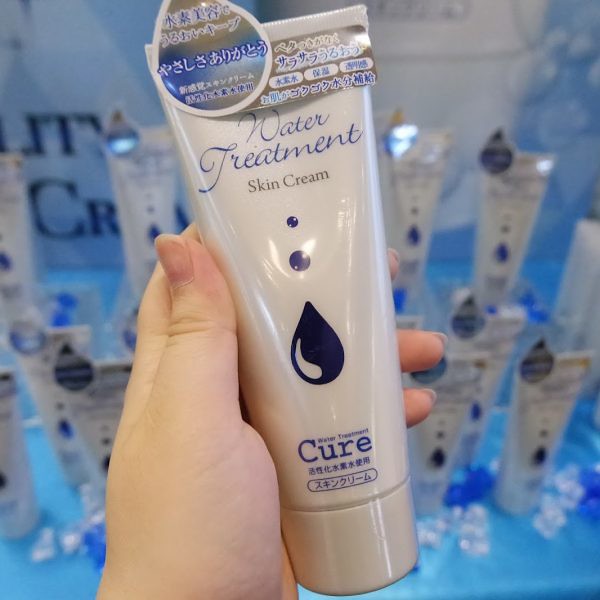This is a horizontally aligned, color photograph with a slight blur, creating a sense of motion or focus on the foreground. The image features a Caucasian female's well-groomed right hand holding a white squeeze bottle of skin cream with a cylindrical cap. The bottle is primarily white and has a triangular shape that widens towards the bottom. Prominently displayed near the top-left, within a magnified circle, are Chinese characters, suggesting an emphasis for advertising purposes. 

The product label features multiple elements: at the top, there's blue and white text over a gold band followed by English text below. The words "Water Treatment" are printed in stylized navy blue cursive on a white background, with an enlarged 'W' and 'T'. Below that, in a more standard font, it states "skin cream." Accompanying the text, there are graphics of blue circular drops and a teardrop-shaped symbol in blue and white. The brand name "Cure" is prominently displayed beneath in bold, blue Times New Roman font.

The background comprises multiple identical bottles arranged in rows, out of focus, within a blue setting reminiscent of both a floor and a wall adorned with scattered white and blue droplets. Additional text in uppercase letters "T-T C-R" appears in dark blue on the upper left side, and on the upper right, there is a large floating white object with a possible seal or lip at the top, framed against white clouds and a blue sky. The overall composition suggests a bright, clean, and cohesive product advertisement focused on skincare.